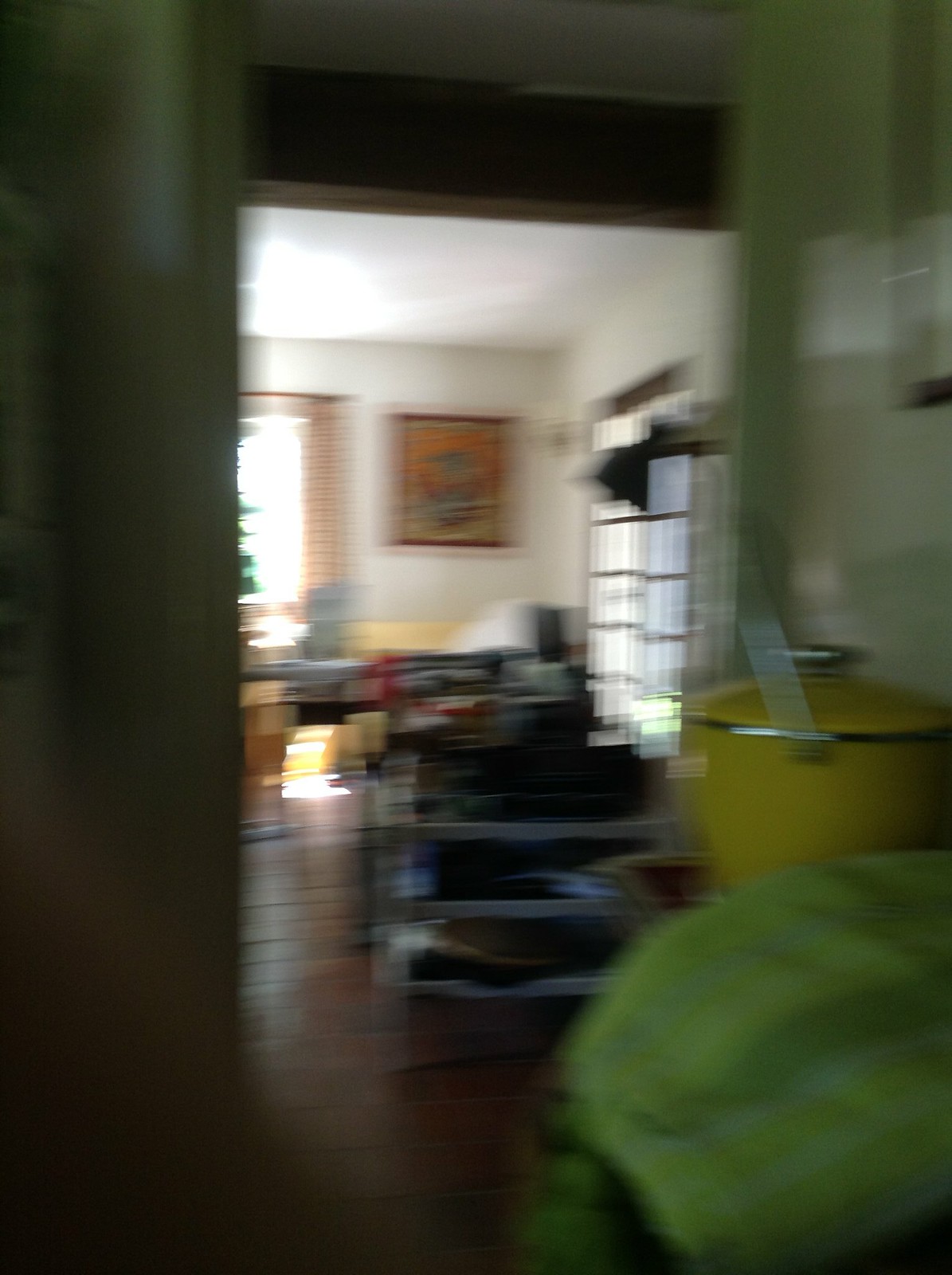In this extremely blurry photograph, we are looking through a cluttered hallway into a brightly-lit living room. The hallway is quite narrow and filled with various items strewn about, creating a sense of disarray. On the bottom right corner, there's a yellow crock pot, while closer to the left side, a light yellowish blanket partially covers some objects on the floor. 

Further into the hallway, which leads directly to the living room, there is a small shelf or shoe rack also cluttered with miscellaneous items. The living room itself is brighter and more spacious, with white walls and wooden flooring illuminated by natural light. To the right side of the living room, there's a window with white curtains featuring black stripes, while another window on the left brightens the space even more.

On the back wall of the living room, there's a picture or tapestry with reddish and yellowish hues inside a brown border. Visible in the living room, albeit unclearly, is possibly a couch, some small boxes, and other assorted objects. The predominant details from all the captions highlight the overall clutter, the bright lighting in the living room, and specific items like the yellow crock pot and the tapestry on the wall.